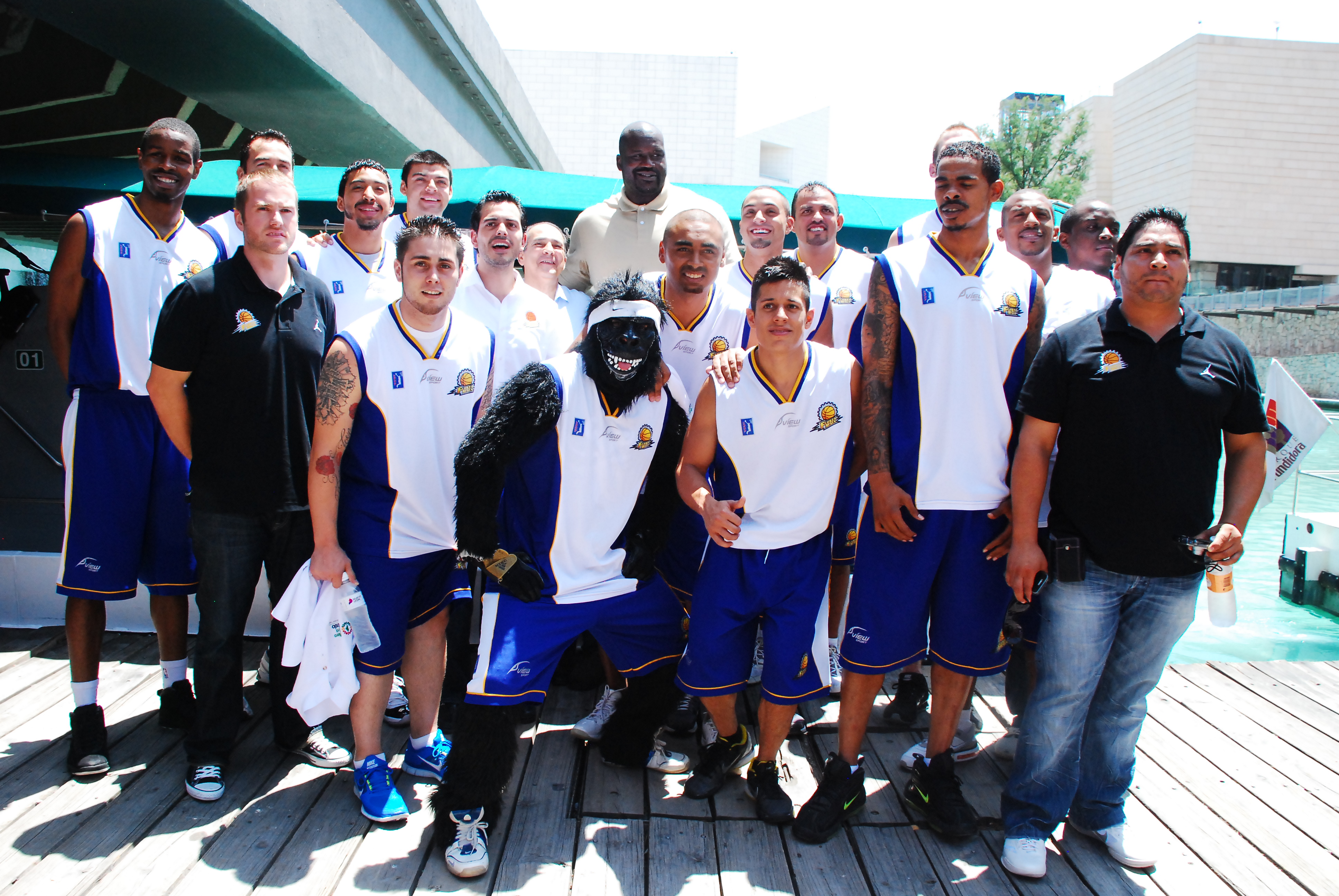A basketball team, featuring around 20 players and two support staff in black polo shirts, poses for a group photo on a light gray, weather-worn wooden dock in front of a light blue body of water. The team members are dressed in a uniform consisting of sleeveless white jerseys with yellow and blue striped collars and blue side panels, along with matching blue shorts adorned with yellow stripes at the hem. Among the standing rows, towering at the back center, is a tall man resembling Shaquille O'Neal, noticeable in his tan polo shirt. Front and center, the team's black gorilla mascot, sporting a giant cartoonish smile and dressed in a basketball outfit, brings a playful energy to the scene. Behind them, crystal-clear water stretches out, with tall buildings, a white structure, and trees dotting the background under a clear sky.